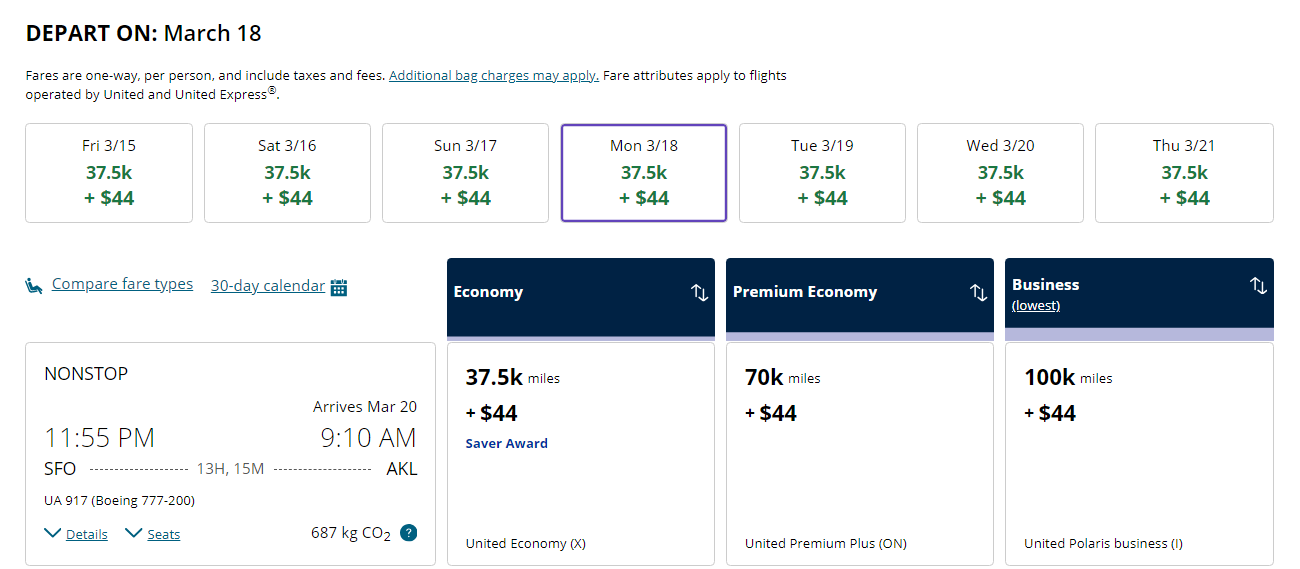A detailed travel itinerary is displayed on a white background. At the top, "DEPART ON: MARCH 18" is prominently written in capital letters. Below this, a note clarifies that fares are one-way per person and include taxes and fees, with additional bag charges possibly applicable. It also mentions that fare attributes apply to flights operated by United and United Express.

Underneath this text, there are seven rectangles, each representing a date and fare cost:
- Friday, 3-15: $37.50 plus $44
- Saturday, 3-16: $37.50 plus $44
- Sunday, 3-17: $37.50 plus $44
- Monday, 3-18: $37.50 plus $44
- Tuesday, 3-19: $37.50 plus $44
- Wednesday, 3-20: $37.50 plus $44
- Thursday, 3-21: $37.50 plus $44

A row beneath these rectangles includes options to "Compare Fare Types" accompanied by an icon of a person sitting in an airline seat, and a "30 Day Calendar" symbolized by a blue calendar icon. 

Further details include a designation for a nonstop flight departing at 11:55 p.m. and arriving at 9:10 a.m. with a note that the arrival date is March 20. The travel route is listed as SFO (San Francisco) to AKL (Auckland), with a flight duration of 13 hours and 15 minutes. The flight is operated by United Airlines, with the flight number UA 917 on a Boeing 777-200 aircraft. Additional icons include a down arrow for "Details" and "Seats," and a carbon emissions estimate of 687 kg CO2, marked with a question mark.

Below the flight information, three fare classes are described:
1. **Economy:** $37.5K miles plus $44 (Saver Reward United Economy X)
2. **Premium Economy:** $70K miles plus $44 (United Premium Plus, marked "ON")
3. **Business:** $100K miles plus $44 (United Polaris Business, indicated as "1")

Each fare class is highlighted with a blue banner box at the top, indicating the respective class names and rewards.